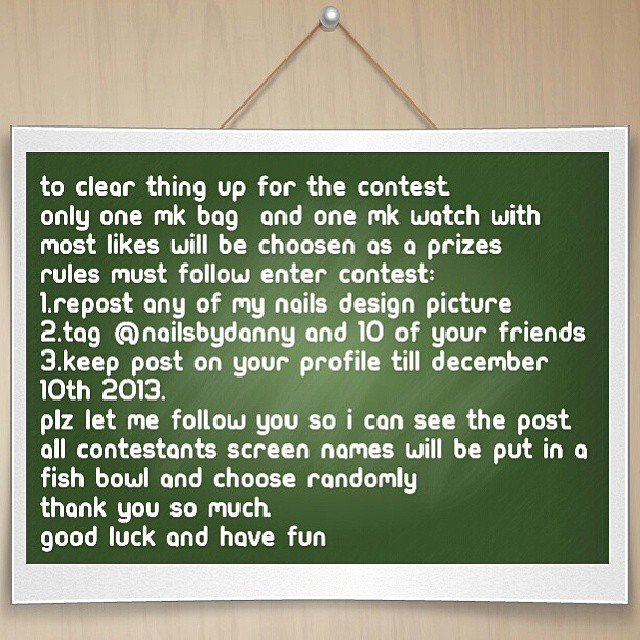The image appears to be a digitally-created graphic resembling a sign hanging on a wall with ropes attached to a pearl pin. The sign has a green background with white text and seems more like computer graphics than a realistic photo. The text on the sign details a social media contest for a chance to win one Michael Kors (MK) bag and one MK watch, each chosen based on the most likes. The rules to enter the contest are: 

1. Repost any picture of the nail designs by "Nails by Danny."
2. Tag "@nailsbydanny" and 10 of your friends.
3. Keep the post on your profile until December 10th, 2013.

Participants must allow "Nails by Danny" to follow them so the posts can be verified. Additionally, all contestants' screen names will be put into a fishbowl, and the winner will be chosen randomly. The message includes several grammatical errors and typos but conveys the essential contest rules and information. The sign concludes with "Thank you so much, good luck, and have fun."